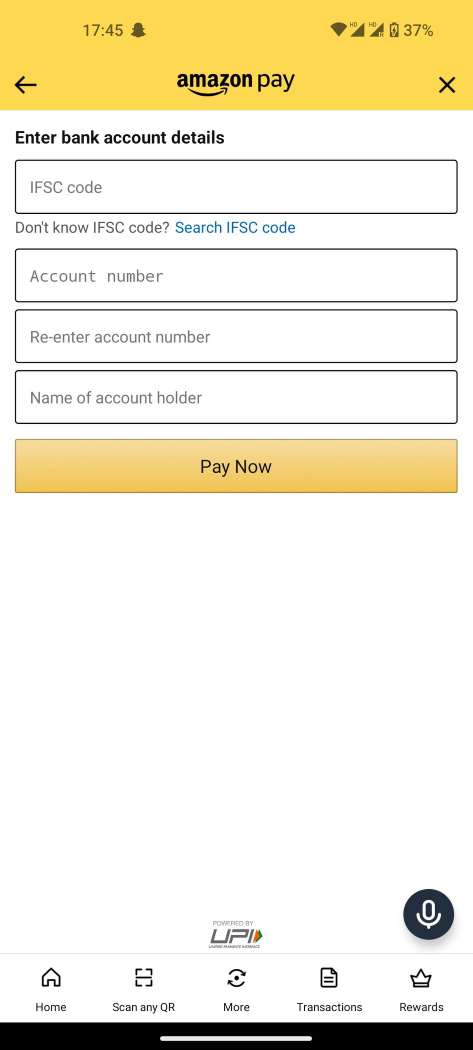At the top of the image, there is an orange box with a black arrow pointing to the left. To the right of the arrow, it displays the time "17:45," followed by icons indicating a notification alert, active Wi-Fi connection, signal strength bars, and a 37% battery level. Below this status bar, there is a header section labeled "Amazon Pay," featuring an "X" icon on the right side for closing the window. 

The background transitions to white where a bold, black text header reads "Enter Bank Account Details." Directly below, there are sequentially organized data input fields, starting with a box labeled "IFSC Code." Followed by a smaller italicized text, "Don't Know IFSC Code" with a blue hyperlink "Search IFSC Code" situated below it for user assistance. The next box prompts for "Account Number," trailed by another labeled "Re-Enter Account Number." Beneath these, there is an input field for "Name of Account Holder." 

At the bottom of this section, an orange button labeled "Pay Now" stands out prominently against some remaining blank space at the footer of the image.